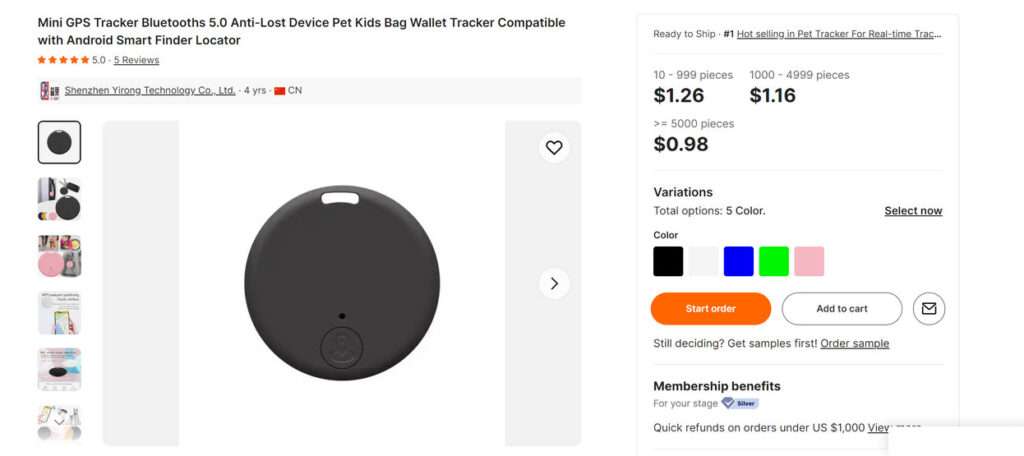The image presents a product listing on a white background. At the top, there's a blue header featuring the product: "Mini GPS Tracker", "Bluetooth 5.0", "Anti-Loss Device", and "Kids Bag Wallet Tracker" compatible with Android Smart Finder Locator. It has a five-star rating based on five reviews. A small blue box, likely representing a technology company, appears next to a red box with "CN" inside it.

On the left side of the image, there are several small pictures arranged vertically. The first picture depicts a black circle inside a box followed by another black circle. The third and fifth pictures show black circles, the fourth and sixth pictures are blurry, and the fifth one has black details in the center. 

A wide blue strip separates these pictures from a large white box showcasing a big black circle with a small white spot at the top. Beneath this, another wide blue strip contains a white circle with a heart at the top and a right-arrow symbol mid-way down.

On the right side, there’s a blue box labeled "Ready to Ship". Below it, different quantity pricing tiers are specified: 10 to 999 pieces at $1.26 each, 1,000 to 4,999 pieces at $1.16 each, and over 5,000 pieces at $0.98 each. 

There are options to select from five colors, indicated by color blocks: black, white, blue, green, and pink. The image prompts users to "Select Now". An orange button labeled "Start Order" and a white button labeled "Add to Cart" are prominently displayed alongside a small circle with an envelope icon indicating "Still Deciding? Get samples first". This is followed by a prompt to "Order a sample" and a section on "Membership Benefits for Your Stage" with a check mark in a blue box, mentioning "Quick Refunds on orders under US $1,000" and an option to "View".